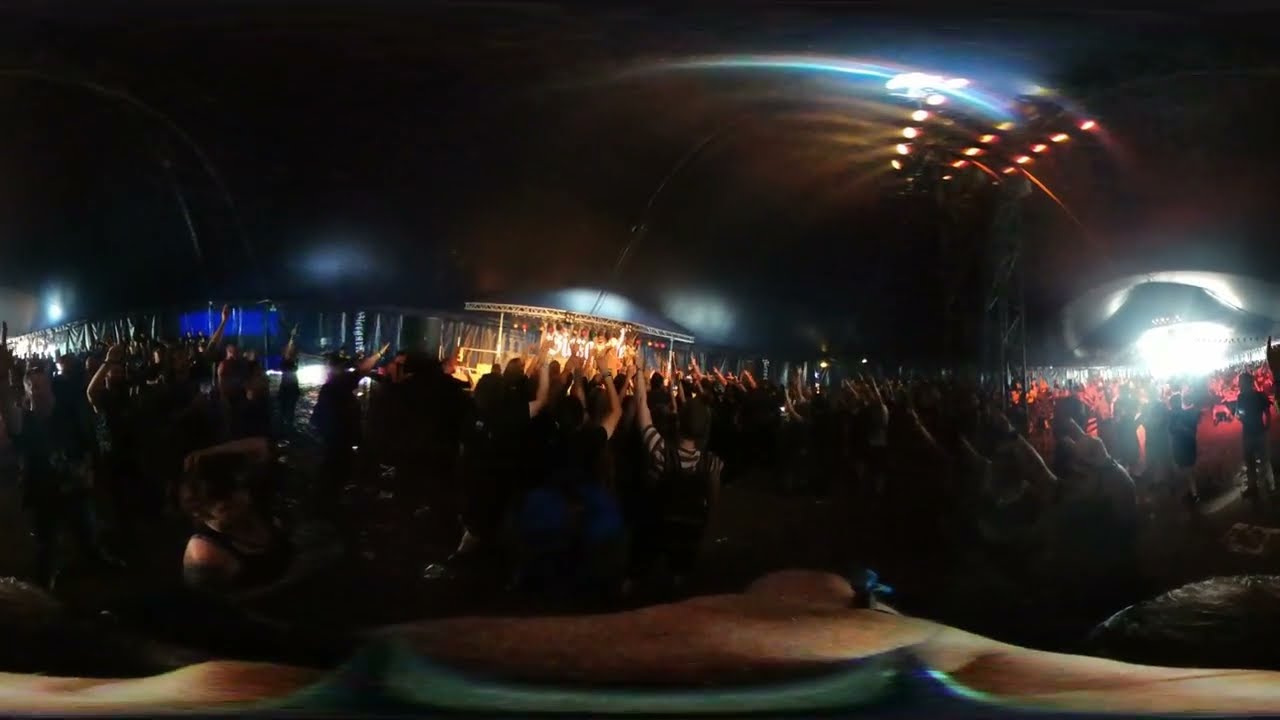The photograph captures a concert held in a vast, packed indoor venue, possibly a stadium, auditorium, or concert hall. The scene is dimly lit, emphasizing the event's intense, electric atmosphere. A sea of people fills the room, all standing with their hands raised in excitement, cheering and directing their attention toward the stage area. Various colored lights — including blue, red, and orange — illuminate the crowd and are emanating from multiple sources, including a prominent, bright light in the top right corner and curved, dotted lights near the ceiling. The wide-angle shot distorts some elements, but it appears there are sections dedicated to stage equipment, including what might be a control setup in the middle and a large screen on the right-hand side to ensure everyone in the enormous hall can fully engage with the performance. The bottom of the photo features an ambiguous, light brown or pinkish form, potentially adding to the chaotic and vibrant ambience of the concert.